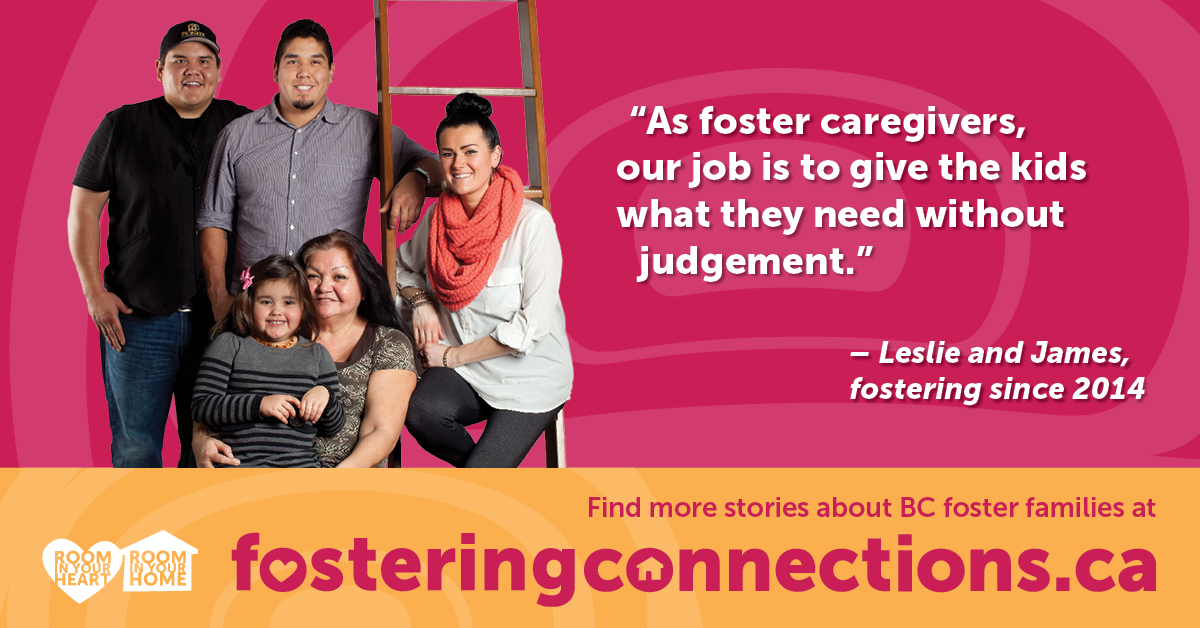The advertisement for fosteringconnections.canada features a vibrant background with hot pinkish-red hues and swirls of lighter pink. To the left side, there is a heartwarming family photo showcasing four adults and one little girl. The family includes a young woman with dark hair tied in a bun, wearing an orange scarf, sitting on a ladder step. An older woman is seated with the little girl on her lap, smiling warmly. Behind them stand two young men. The text to the right of the image states, "As foster caregivers, our job is to give the kids what they need without judgment. Leslie and James fostering since 2014." At the bottom, a yellow banner with lighter yellow swirls reads, "Find more stories about BC foster families at fosteringconnections.ca." Additionally, there are small icons to the left featuring a heart and house with the messages, "Room in your heart" and "Room in your home."